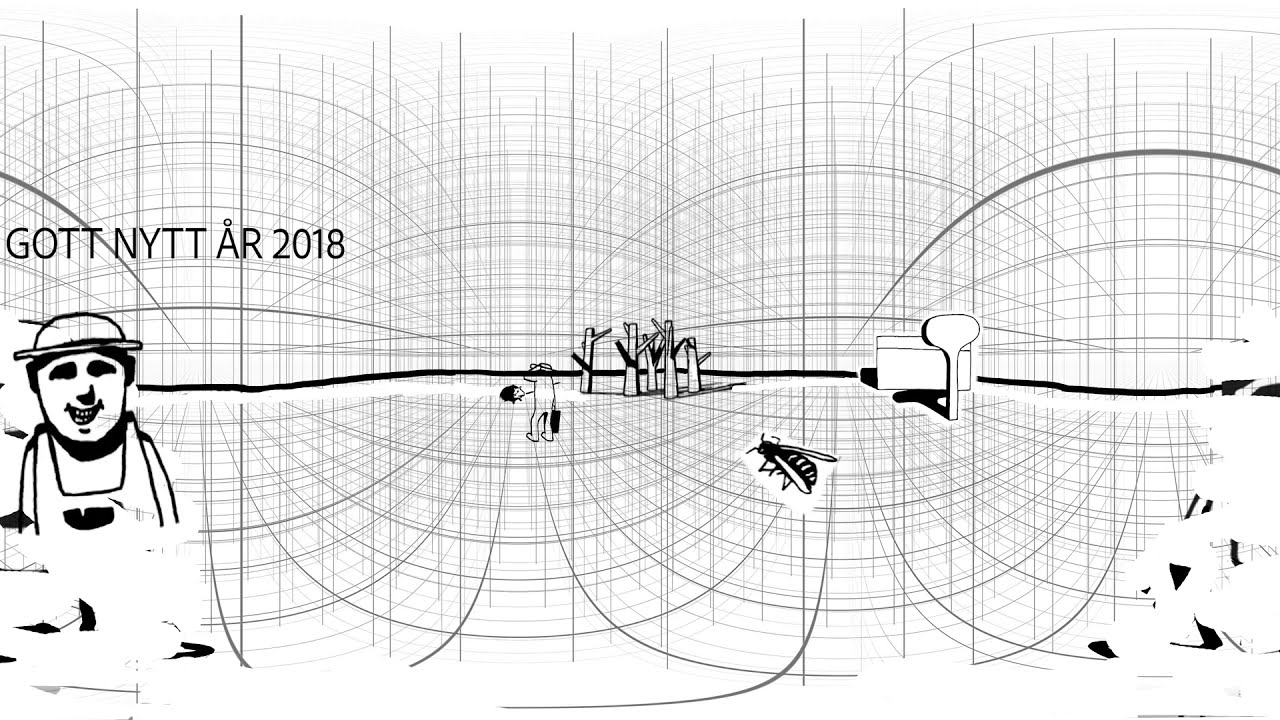A detailed black and white illustration features a surreal, panoramic scene dominated by intricate circular and curved lines forming a grid-like pattern with hemispherical arcs that warp the horizon. A bold, black horizontal line runs across the center, dividing the sky from the ground. This surrealistic image includes a variety of elements: to the left, a rudimentary cartoon figure wearing a bowler hat and apron smiles, reminiscent of an old-time farmer, with the text "GOTT NYTT AR 2018" above it. In the center, a small cluster of barren, leafless tree stumps stands, overshadowed by a large, detailed black and white bee. To the right, a vacant white building with an adjacent water tower completes the eerie but fascinating landscape.